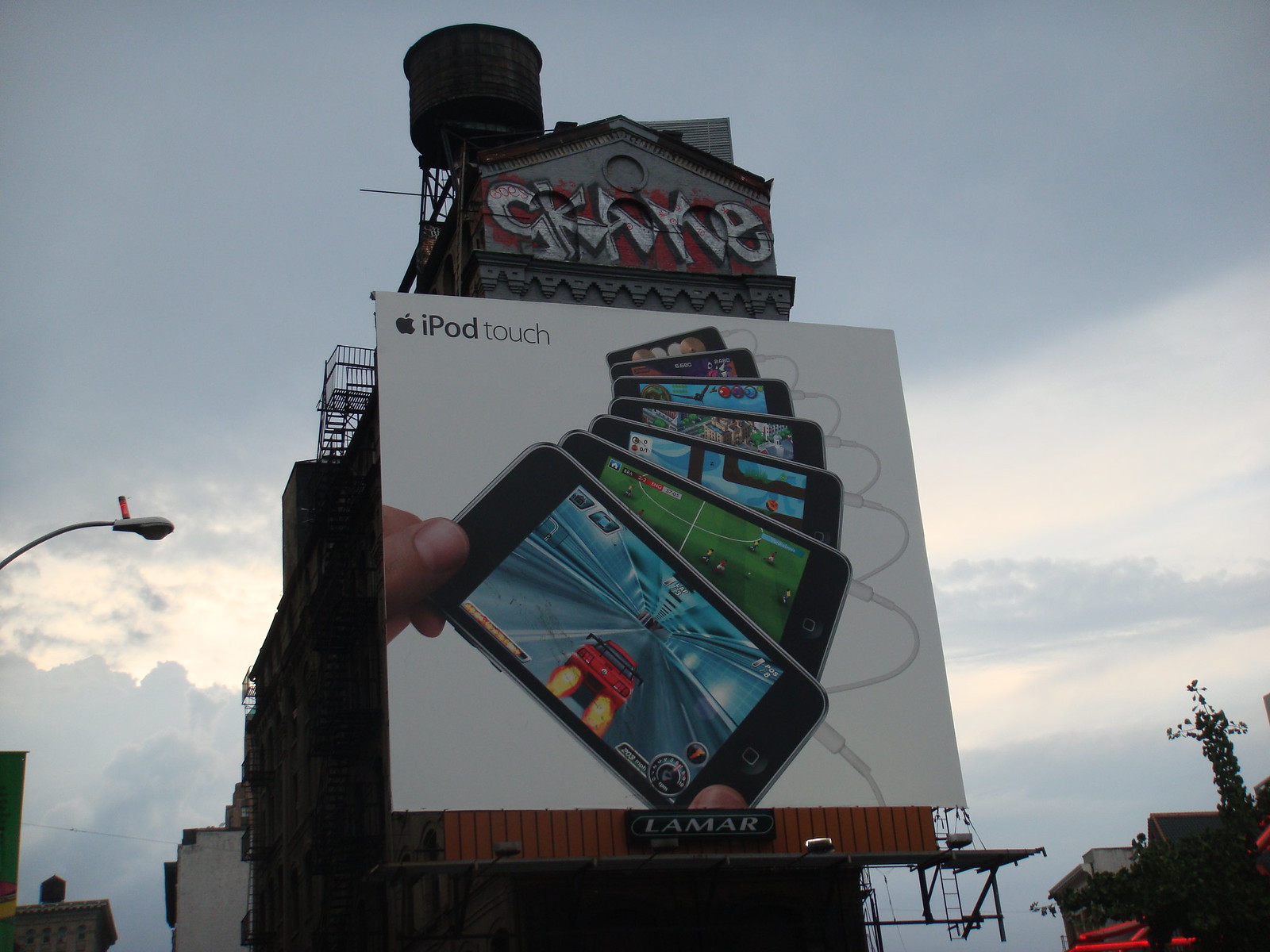The photograph depicts a large, outdoor billboard taken during the day. The billboard is square and prominently features Apple branding in the upper left corner, displaying the black Apple logo alongside the text "iPod Touch." The focal point of the billboard is an image of a thumb and forefinger holding an iPod, which is slightly tilted downward to the right and has a white charger plugged into it.

Surrounding the foreground iPod are six other iPhones, fanned out like a deck of cards from the top of the iPod. These iPhones show only about a third of their screens, each displaying different, vividly colored screen images. The background of the image reveals a clear sky with some gray and white clouds, adding a touch of natural scenery to the tech-focused advertisement.